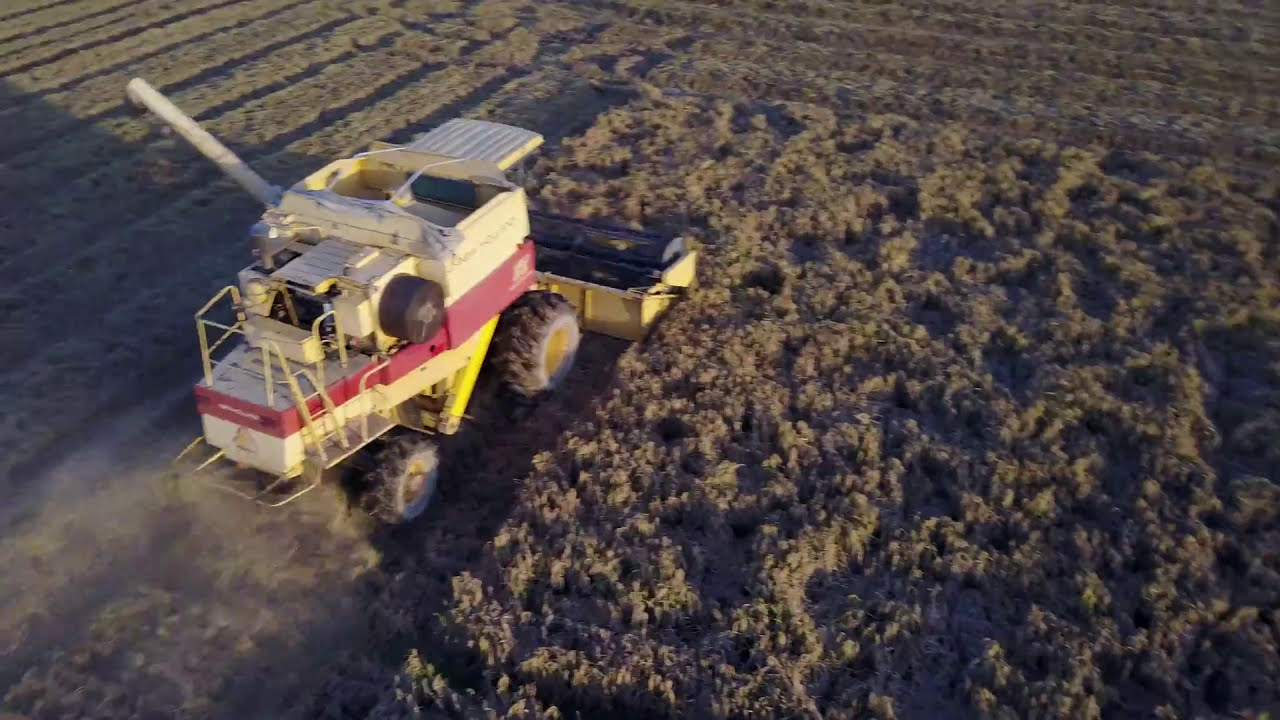In this color landscape drone photograph, a large tractor is depicted working in a vast farmland field. The tractor, predominantly white with a distinctive red stripe and some yellow areas on the bottom, features big black wheels. It is centrally placed towards the left of the image, moving in a southerly direction towards the bottom left corner. The vehicle appears to be engaged in harvesting or plowing, as evidenced by a yellow-black section projecting out and either cutting down or gathering the crops, creating a dusty, yellowish haze behind it. Surrounding the tractor is an expansive field characterized by a mix of brown and deep green crops, organized in neat, rectangular rows. The field on the right is filled with dark green olive-colored vegetation, while the rowed plants lie on the left. Despite the visible dust, no text can be clearly read on the tractor due to its blurriness. Overall, the photograph showcases a realistic, representational depiction of agricultural activity from an aerial perspective.